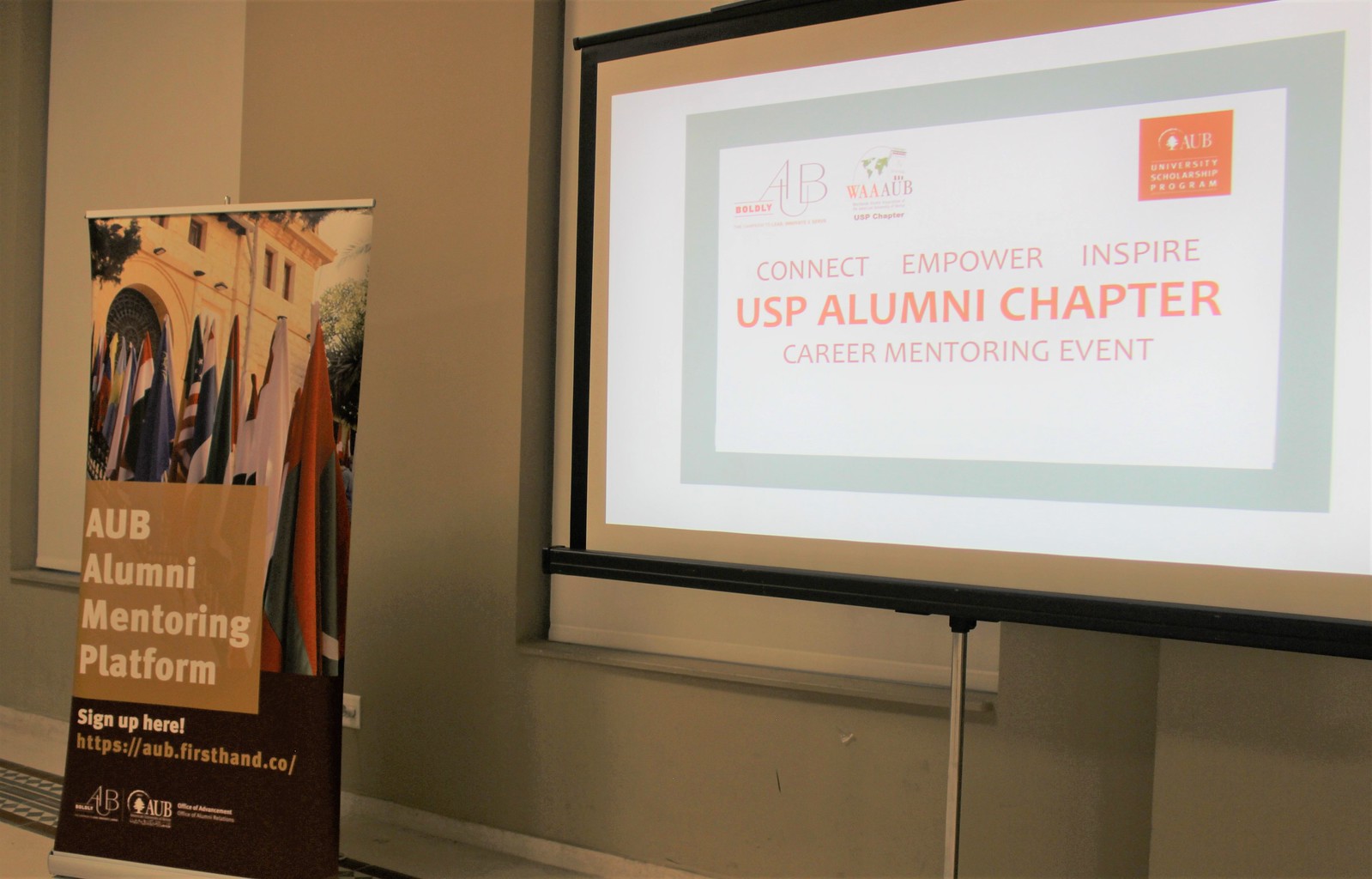The image depicts a projected PowerPoint slide on a wide white rectangular screen, located on the right side of a light gray-walled room with two windows covered by blank white blinds. The slide itself features a white background with a small light blue frame, containing a central section with a sage green rectangle border. Inside this border is an orange square positioned in the upper right corner that displays a logo and text. The main body of the slide is center-justified and reads "U.S.P. Alumni Chapter Career Mentoring Event" in orange font. Above this text, keywords state "Connect, Empower, Inspire." To the left of the projection, there is a prominent standing sign positioned between the windows, displaying an image of several flags in front of a brown building, with text that reads "AUB Alumni Mentoring Platform" and a prompt to "sign up here."